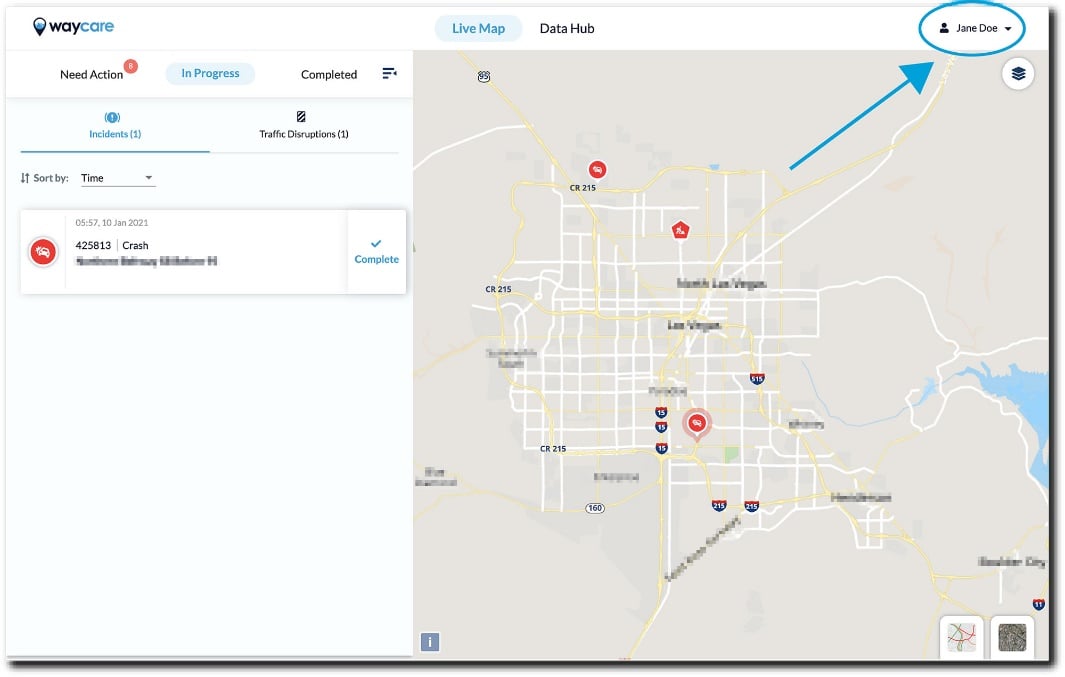The image is a screenshot bordered with a light gray rectangular frame. In the upper left corner, “Wacare” is prominently displayed in black and blue text. Adjacent to this, a blue box contains the words “Live Map,” and to the immediate right, “Data Hub” is written in black text. The upper right corner is marked by a blue circle highlighting “Jane Doe,” with a blue arrow pointing to it. 

On the upper left side, the text “Need Action” appears in black, followed by “In Progress” in blue, and “Completed” in black. Beneath these labels, the section continues with blue text reading “Incidents 1,” “Traffic Disruptions 1,” and “Sort by Time,” next to a pull-down menu. 

Below this section, an entry dated “10th of January, 2021” at “5:57” is documented. A red circle with an icon of a crashed car is prominently featured. To its right, the description “425, 813, Crash” is present, and further right, the status reads “Complete” in blue text accompanied by a check mark.